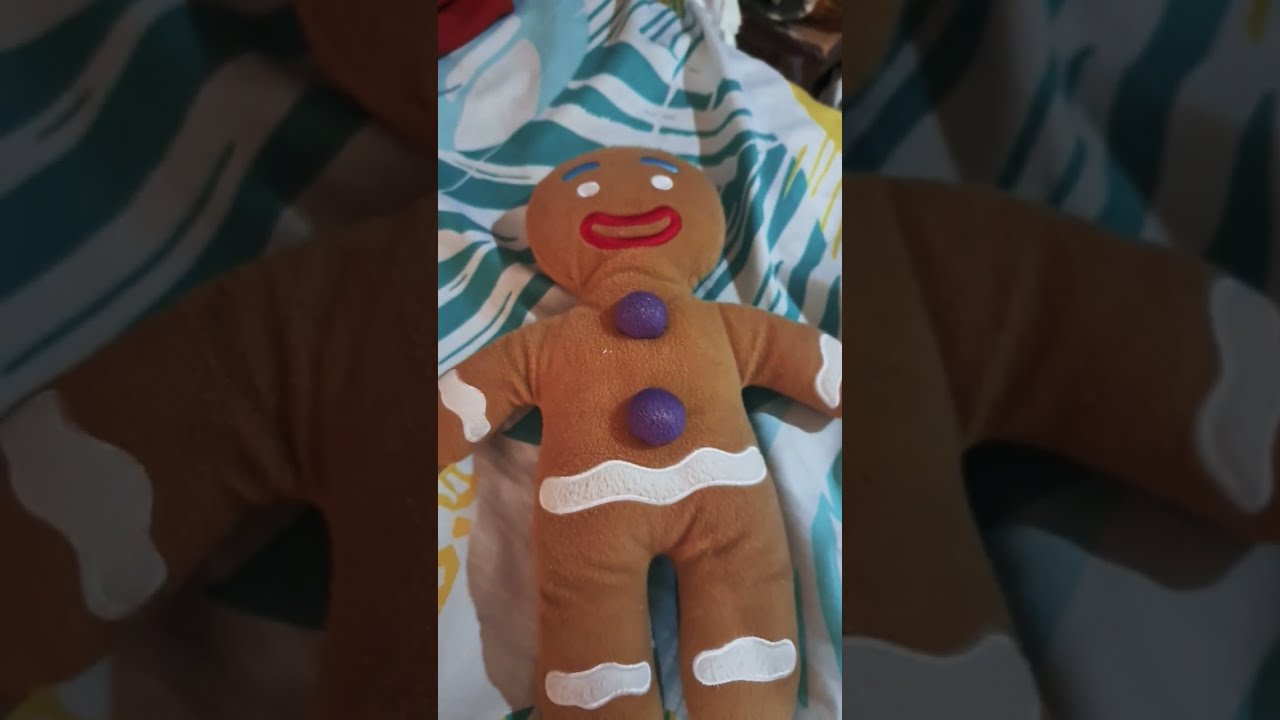In a unique composition featuring a photograph within a photograph, the central image is brightly highlighted while the surrounding background image is faded and more blackened. The focal point of the central image is a gingerbread man plush toy laying atop a vividly patterned blanket. The gingerbread man is light brown, resembling fleece fabric, and details like white frosting lines accentuate his arms, waist, and legs. He has cheerful light blue eyebrows, white eyes, and a red-outlined smiling mouth. Decorating his torso are two purple pom-poms serving as buttons. The soft textures and colors of the plush contrast with the intricate blanket it rests upon, which features a predominantly white background interlaced with dark green, light blue, and yellow stripes, adding a colorful and cozy ambiance to the scene. The entire composition suggests an indoor setting and captures a still moment, possibly extracted from a video, with the central image prominently displayed against its muted duplicate in the background.